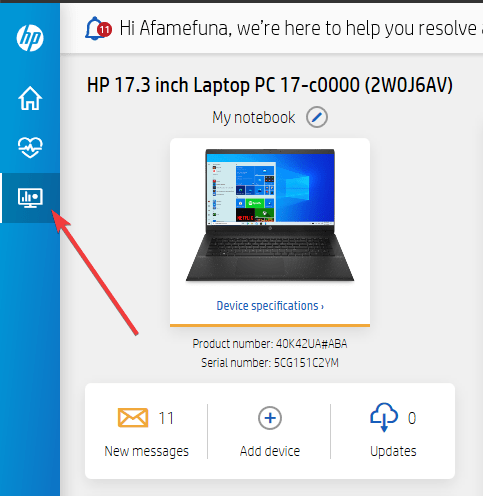The image displays a detailed interface of an HP 17.3-inch laptop PC, model 17-C0000, titled "My Notebook". A prominent blue bar runs vertically down the left side. At the top of this bar is a circle containing the letters "HP", followed by an icon of a simple house outline, symbolizing the home screen. 

Beneath the house icon is a heart symbol, pierced by a heartbeat line, likely indicating health monitoring or system status. Next is the image of a computer monitor with an arrow pointing towards it, possibly representing device focus or screen activity.

In the upper-right corner of the image, there is a notification bell featuring a red badge with the number 11, signaling new alerts or messages. A greeting text starts with "Hi, amifamifun, we're here to help you resolve", but is cut off.

Further down, the image showcases detailed device specifications, including the product and serial numbers, with a labeled section beneath stating "Device Specifications". Below this is a wide white bar divided into three sections by two gray lines. 

The first section displays an envelope icon with the number 11 beside it and "New Messages" underneath, indicating unread messages. The middle section shows a gray circle with a blue plus sign, labeled "Add Device", suggesting the option to connect additional devices. The final section features a blue cloud icon with an arrow pointing downwards, labeled "Updates", referring to pending software or system updates.